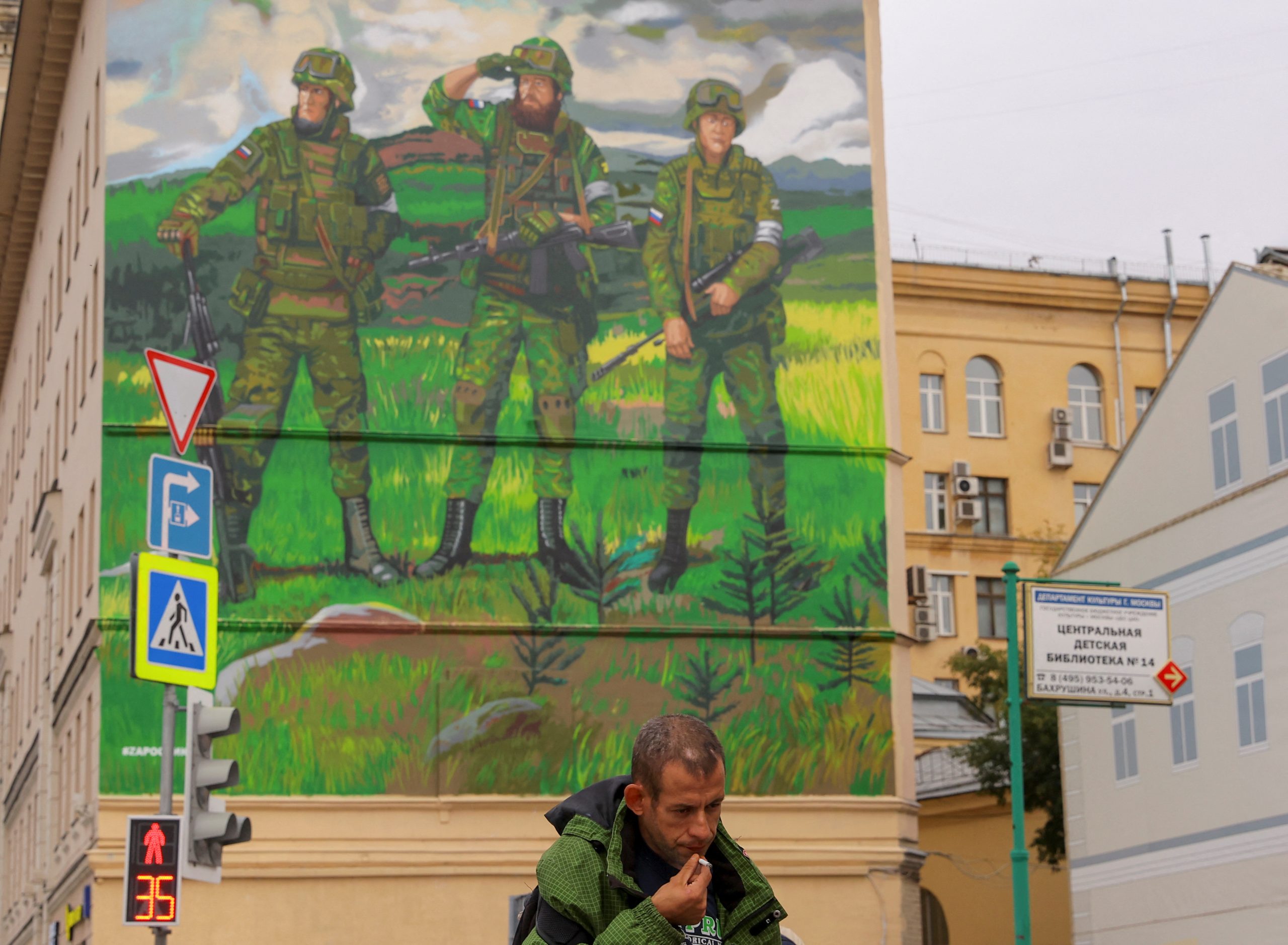The photograph, taken outdoors under a light gray sky, meticulously captures an urban scene framed by various street signs and architectural details. Dominating the right side is a white, three-story residential building, complemented in the background by a five- to six-story yellow apartment complex. Prominent in the scene is a large, detailed mural on a building’s façade, depicting three soldiers in green camouflage standing in a vibrant green meadow with flowers. Each soldier grips a firearm—a rifle, one of them saluting. The soldier on the left gazes leftward, while the soldier in the middle shields his eyes from the sun, and the soldier on the right looks in the opposite direction of the others. Below this mural stands a man in a green jacket accentuated with black, smoking a cigarette. He has short black hair and a receding hairline. Close to him are several street signs and traffic signals, including a red pedestrian signal with illuminated numbers "35," various directional signs, and a walking symbol. A mix of residential buildings flanks the mural, enriching the cityscape. The writing on some signs appears to be in Russian, further grounding the photograph in its locale.